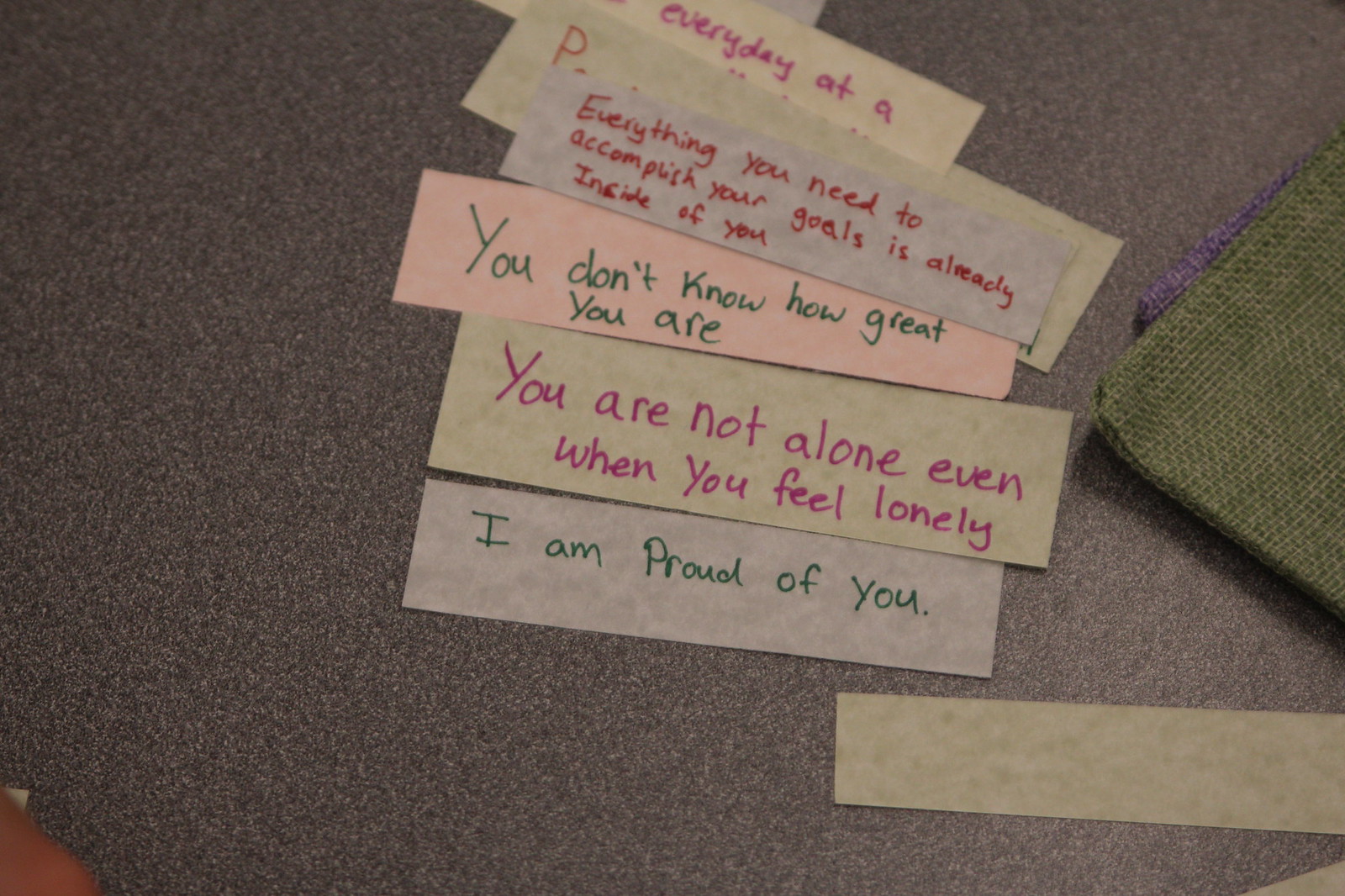The photograph captures an arrangement of rectangular paper strips with inspirational sayings, laid out on a gray surface that resembles a salt-and-pepper granite countertop. The surface is textured with a static gray and white pattern. The paper strips, which are similar in size to those found in fortune cookies, vary in color, including shades of off-yellow, gray, and pink. Each strip features handwritten text in marker. Among the visible messages, one strip reads, "Everything you need to accomplish your goals is already inside of you." Below it, another says, "You don't know how great you are." Further down, the strips proclaim, "You are not alone even when you feel lonely," and "I am proud of you." To the right of the paper strips, a green woven piece of fabric, possibly a placemat or napkin, is partially visible, with a hint of a purple fabric layer underneath. In the bottom right corner, there is an off-yellow blank strip of paper. The strips are placed closely together, some stacked on top of others, creating a layered effect.